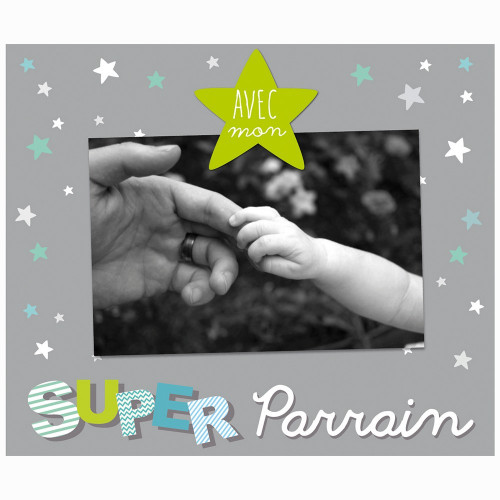This image appears to be a greeting card featuring the words "Avec Mon" in cursive at the top, accompanied by a green star. It showcases a black and white photograph centered on the card, where a child's hand reaches to hold the finger of an adult hand, which is adorned with a ring. Adding a lively touch, the card is framed with a wide gray border decorated with green, white, and gray stars. Along the bottom, the words "Super Parrain" are creatively displayed, with the "S" featuring blue and white stripes, the "U" in green, and varied designs filling the other letters. This card seems to convey a heartfelt message, possibly celebrating a birth or showing appreciation, with a touching, star-studded design around the central image.